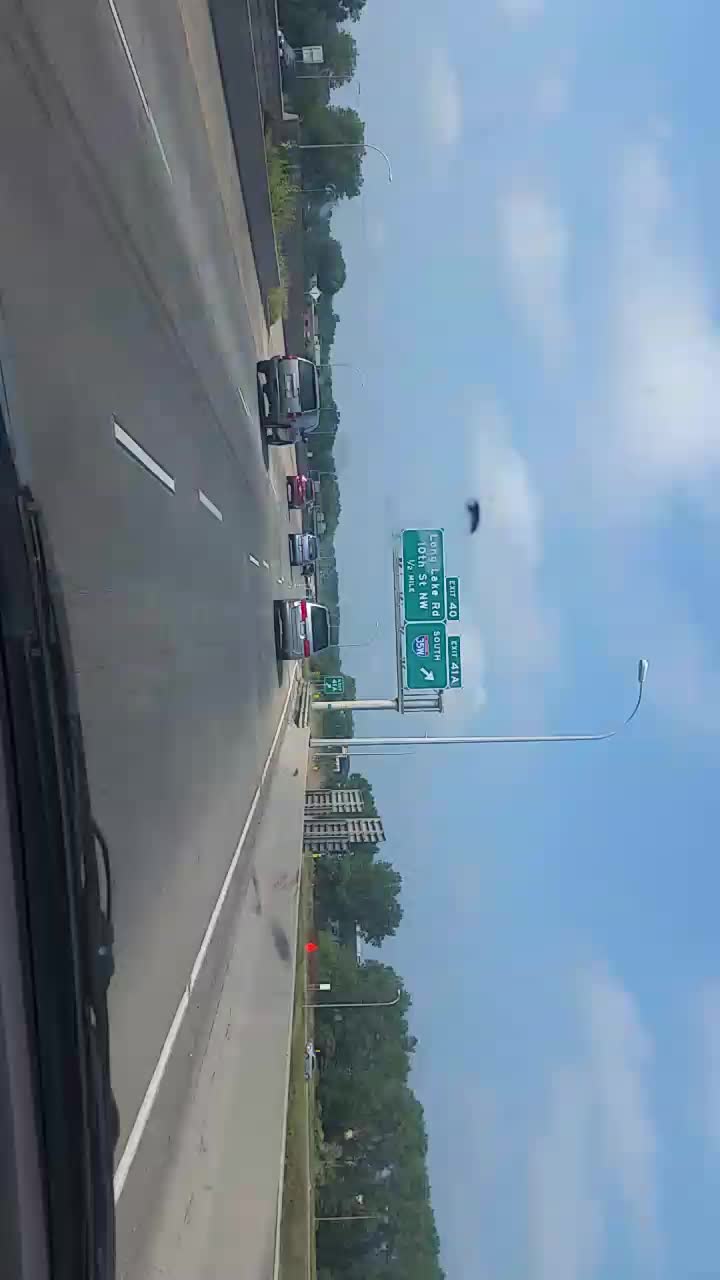This high-resolution photograph, taken from inside a vehicle, captures a moment on a bustling highway. The viewpoint reveals parts of the vehicle’s black windshield wipers and gray dashboard. The smooth black pavement of the highway is marked with crisp white lane dividers and a solid white line at its edge. Overhead, green road signs, adorned with clear white fonts and directional arrows, guide the way. A variety of vehicles populate the scene, including a silver van, a white-gold van, a red car, and a silver car, all traveling along the highway.

The backdrop features a picturesque blue sky filled with fluffy white clouds and verdant, leafy trees lining the roadside. A white pole stands visible against this scenic backdrop. In the distance, additional road signs and a metallic structure are also discernible, adding to the depth and detail of this crystal-clear highway scene.